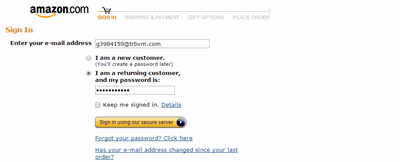This is a detailed and descriptive caption for the provided image:

The color screenshot appears to be taken from Amazon.com, featuring the distinct Amazon.com logo in the top left corner. The logo displays 'Amazon' in darker bold text, while '.com' is written in a slightly lighter black. The signature A to Z arrow, colored yellow, points from the letter 'A' to 'Z' beneath the text.

The page depicted is a sign-in screen. At the top, there is a 'Sign-In' button accompanied by a shopping cart icon. Next to these, there is a set of navigation options including 'Shipping and Payment', 'Gift Options', and 'Place an Order'. Prominently, the page displays the title 'Sign-In' in orange, matching the hue of the yellow arrow under the logo.

An instruction to 'Enter your email address' appears above a text box where the user has input their email, albeit slightly blurred, appearing as G3964159@BRBVM.com. Below this, there are two options: One for new customers to create a password later and another for returning customers to enter their existing password. The returning customer option is selected, and a password has been entered, though it is obscured by dots for security.

Further down, there is a checkbox for 'Keep me signed in' and a button labeled 'Sign-In using our secure server'. Below these options, links for 'Forgot your password? Click here' and 'If your email address has changed since your last order' are available for additional account recovery and update options.